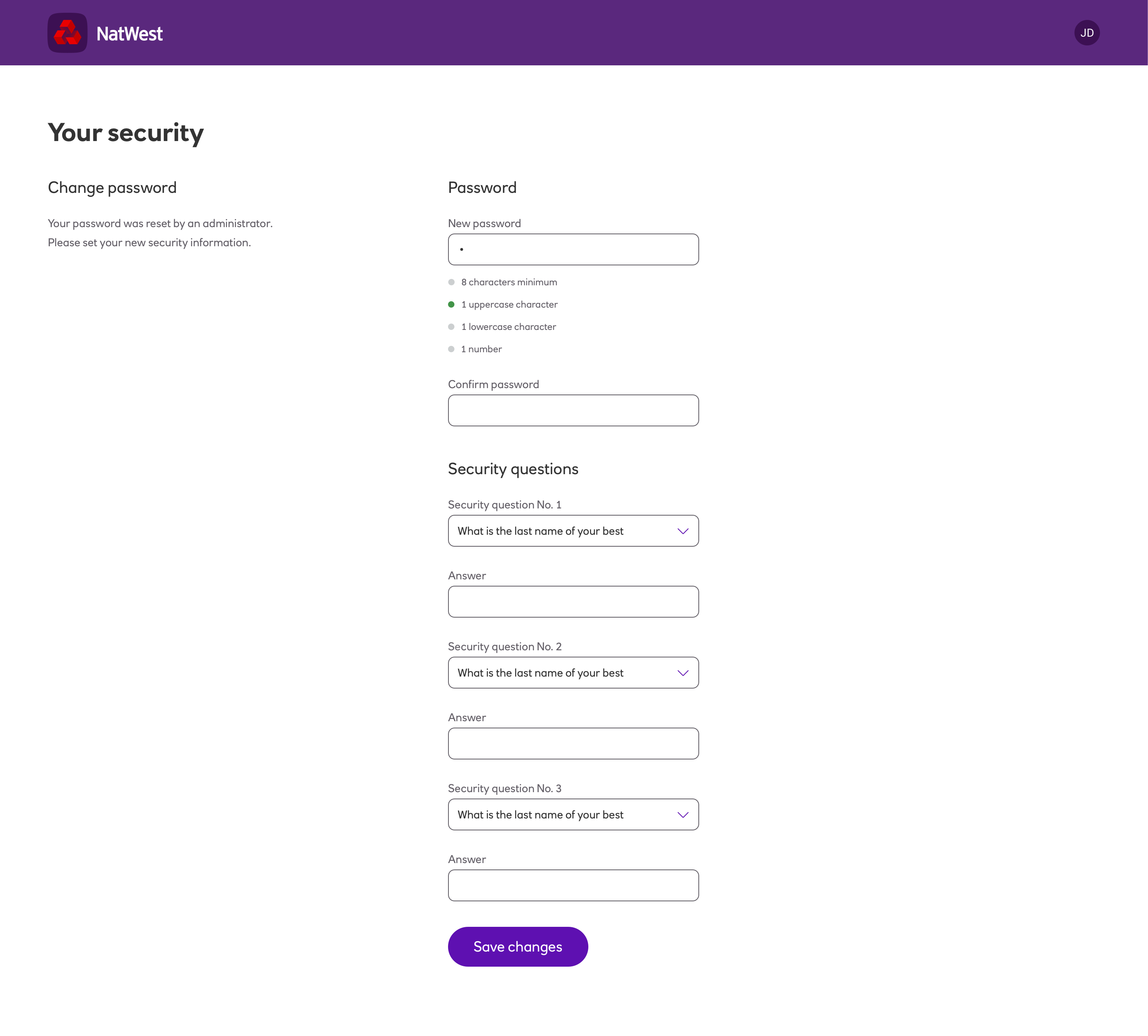The image is a screenshot of a "Change Password" page from the NatWest website. At the very top, there is a dark purple bar, with the NatWest logo located on the left side, featuring the text "NatWest" in white alongside three red cubes arranged in a triangle. On the right side of this bar, there is a dark purple circle containing the initials "JD".

Beneath the purple bar, a large white box occupies most of the screen. On the left, bold text reads "Your Security" followed by "Change Password," indicating the purpose of the page. An informative message below states, "Your password is reset by an administrator. Please set your new security information."

On the right side of this section are input fields labeled "Password" and "New Password". The new password input field currently has one character entered and includes requirements like eight characters minimum, one uppercase character, one lowercase character, and one number. The criteria for "one uppercase character" is highlighted, indicating it has been met.

Below the "New Password" field, there is a "Confirm Password" input box to verify the new password. Following this, in bold black font, the page displays "Security Questions." For Security Question 1, the dropdown menu reads "What is the last name of your best?” with an answer input box provided. The same security question and answer format is repeated for Security Question 2 and Security Question 3. 

At the bottom of the page, there is a prominent purple button labeled "Save Changes".